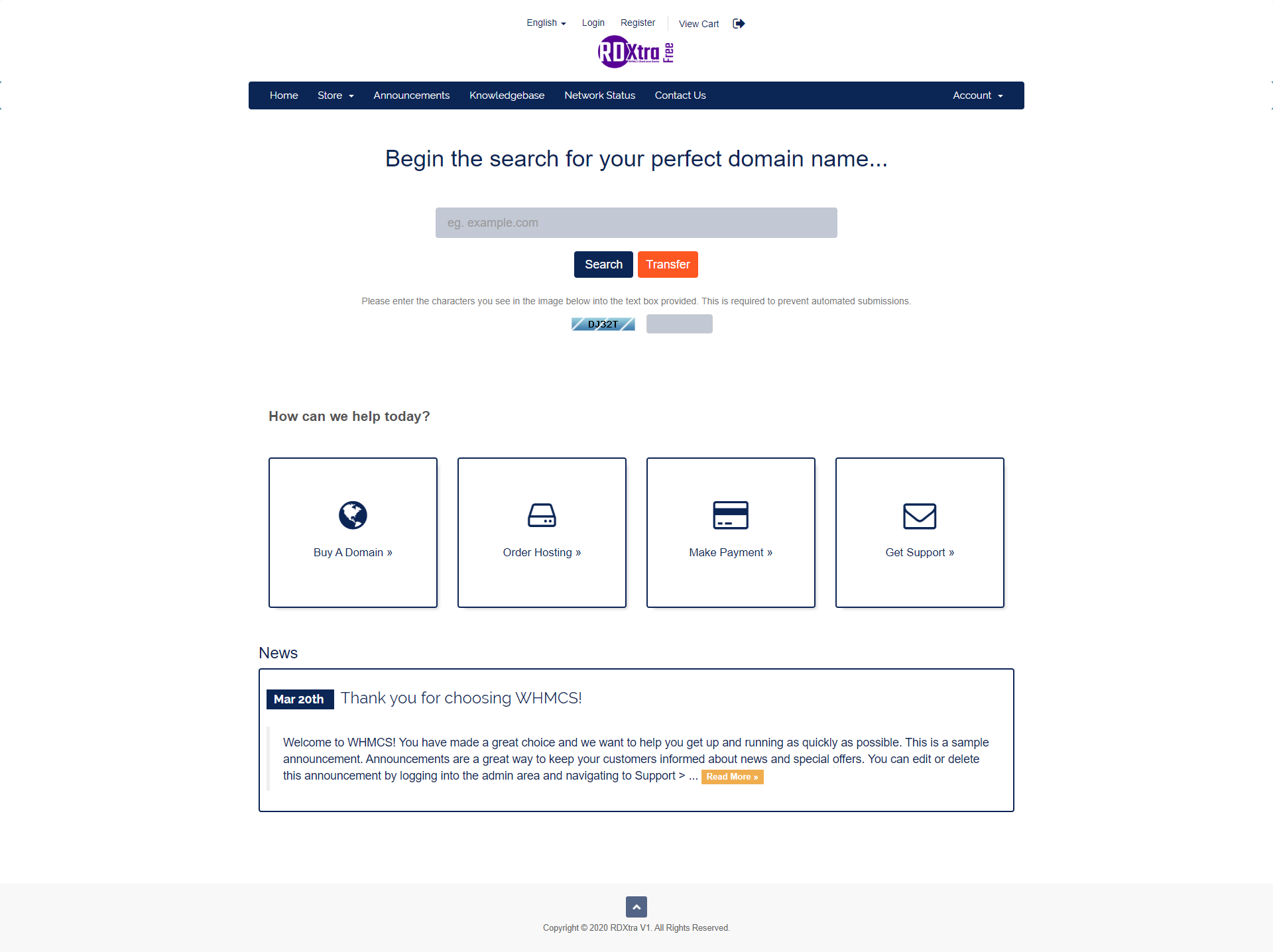The caption describes a detailed view of a website's homepage, evidently for a service named RD Extra, offering domain registration and related services. Here's a refined and detailed description for the screenshot:

---

The screenshot depicts the homepage of a web service named "RD Extra." The page prominently features the logo "RD Extra" with the word "FREE" immediately following it. At the top of the page, there's a navigation bar with various options, including language selection, "English," and links to "Login," "Register," "View Cart," and a right-arrow icon.

Below this, a top banner consists of several buttons labeled: "Home," "Store," "Announcements" (with a drop-down menu), "Knowledge Base," "Network Status," "Contact Us," and "Account" (also accompanied by a drop-down menu).

Central to the page is a bold message inviting users to "Begin the search for your perfect domain name," alongside a search box pre-filled with "example.com" and buttons labeled "Search" and "Transfer." Just below this search section, there's a CAPTCHA prompt instructing users to enter characters to prevent automated submissions.

In the middle section of the screenshot, the text "How can we help today?" is displayed, with several action buttons underneath, including "Buy a Domain," "Order Hosting," "Make a Payment," and "Get Support."

A news update dated March 20th includes a welcoming message: "Thank you for choosing WHMCS!" The announcement welcomes users to WHMCS and reassures them of support in getting started quickly. This sample announcement explains the usefulness of such posts in keeping customers informed about news and special offers. It mentions that announcements can be edited or deleted from the admin area under Support.

Overall, the webpage has an informative and navigable layout, featuring numerous buttons for assistance and support set against a white background, anchored by the RD Extra/free logo.

---

This detailed caption covers the essential elements and user interface details described in the original voice input.